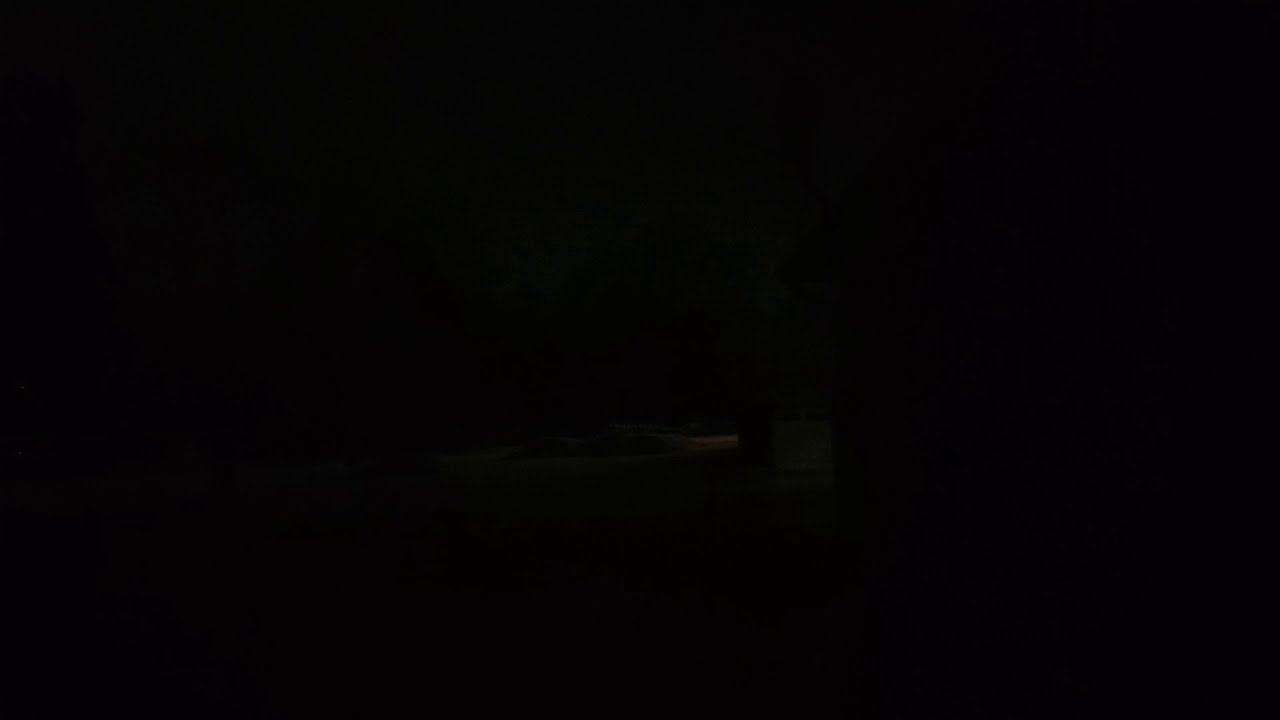In this image, we see a predominantly black background, creating a dark and ambiguous scene. At the center, there is a small, light-colored area, tinged with a very light shade of pink. The scene appears to depict a 3D object that is difficult to identify, possibly resembling a missile or a car, and is likely taken at night. The setting may include elements suggestive of a garage and a road, with the night sky overhead. The screenshot seems to be taken from some kind of application, capturing an obscure figure within an entirely black backdrop.